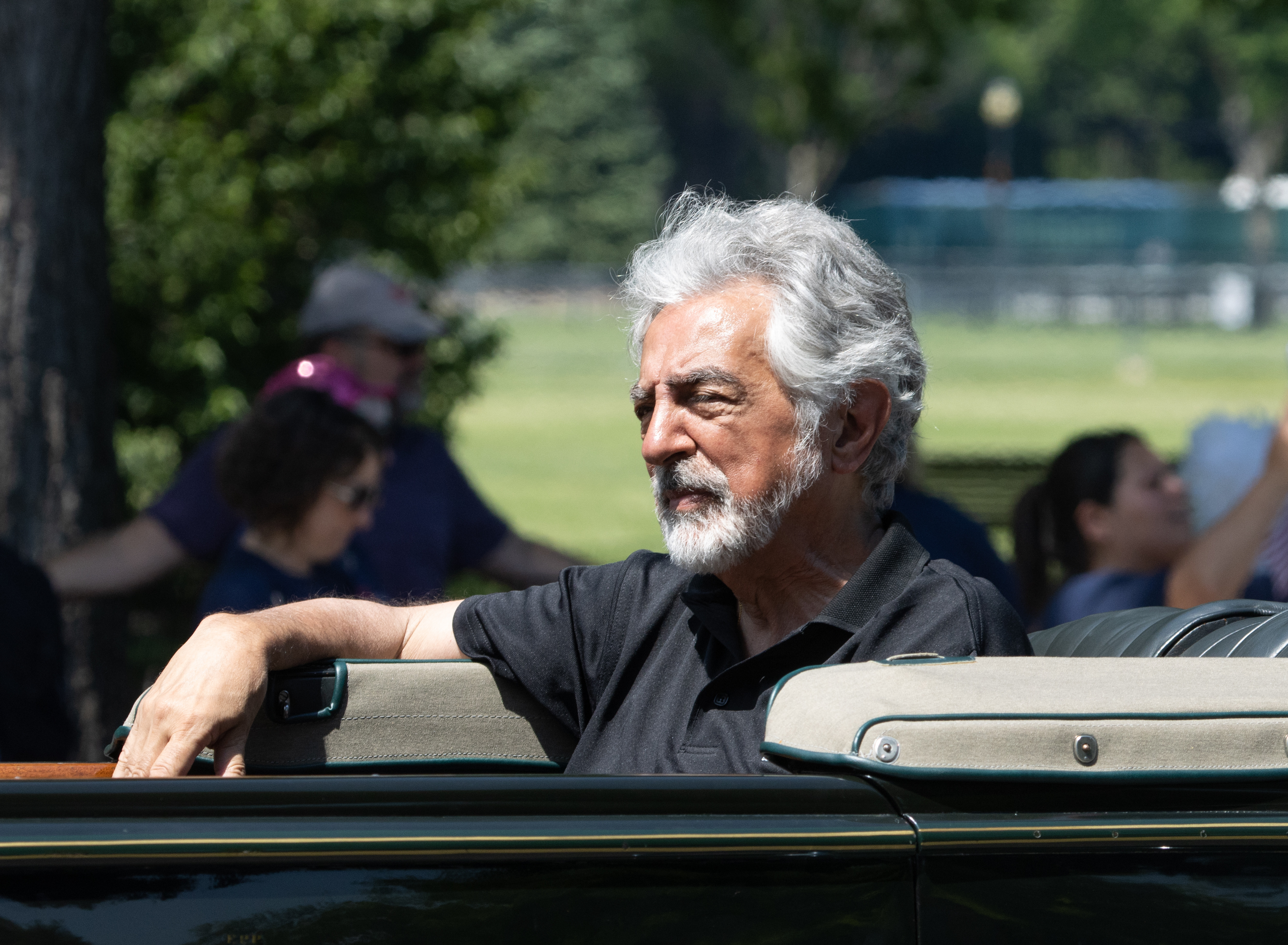In this vibrant color photograph, an older man with shaggy white hair, a matching beard and mustache, and tanned skin, sits in a black convertible adorned with gold trim at the top. He wears a black polo shirt with short sleeves that reach the middle of his biceps and two buttons casually undone. Resting his arm on the side of the car, he squints his eyes, suggesting sunlight. The car features black leather seating and a large bench seat in the back, partially visible as the car's edges are cut off by the photo's frame. 

Behind the vehicle, a blurry yet detailed scene unfolds. A baseball field with lush green grass stretches out, enclosed by a chain-link fence and bordered by a verdant tree line in the far background. Multiple people populate this backdrop. To the right of the man in the car, one woman with a ponytail and blue shirt appears to have her arm raised, while to the left, a man and a woman, both in dark blue shirts, stand together. The man sports a baseball cap and sunglasses, and the woman, who has short dark hair, wears sunglasses. Another figure behind them, possibly a man, is distinguished by a purple scarf. This bustling scene offers a glimpse into a lively outdoor setting on a sunny day, with everyone seemingly drawn to an unseen event or activity off to the right.